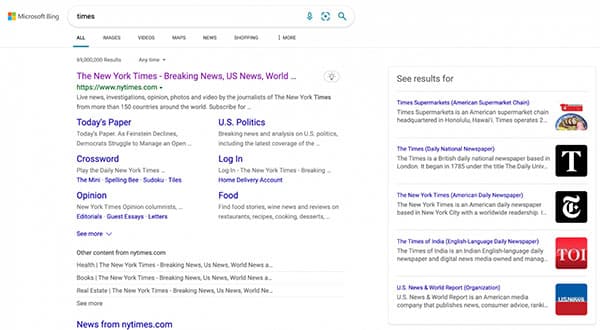In this image, which appears to be a screenshot of a computer search, the background is predominantly white. In the top left corner, "Microsoft Bing" is displayed in small, bold, gray font, alongside the Microsoft logo, which consists of four small squares arranged to form a larger square. The logo features the colors red, green, blue, and yellow.

In the search bar next to the logo, the word "Times" is typed in black font. Below the search bar, there is a navigation menu with various options like "All" (selected and underlined in blue), "Images," "Videos," "News," "Maps," "Shopping," and an additional option.

The first search result appears to be selected, shown in large purple font. It reads: "The New York Times - Breaking News, U.S. News, World..." followed by the URL "https://www.nytimes.com" in black font. Below this link, there are sections for easy navigation, starting with "Today's Paper" in blue font, and underneath it, options for "Crossword" and "Opinion." Adjacent to "Today's Paper," there are links for "U.S.," "Politics," "Login," and "Food."

On the right-hand side of the image, there is a separate box outlined in thin gray lines. At the top left of this box, it reads "See Results For," followed by clickable options such as "Times Supermarket," "The Times Daily," and "National Review Paper."